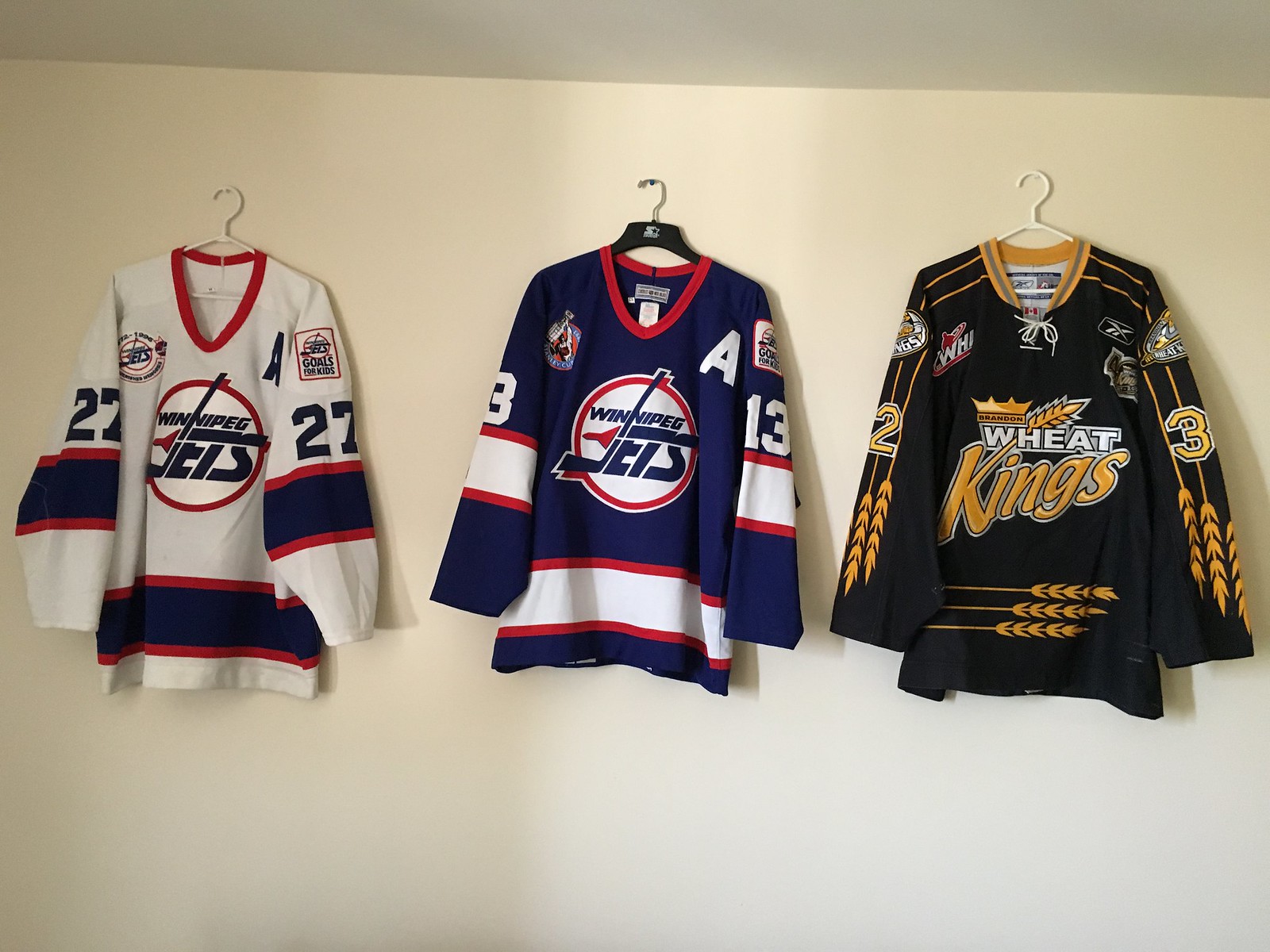The photograph showcases three hockey jerseys hanging on a light gray wall, just a few inches below the white ceiling. The leftmost jersey is a predominantly white Winnipeg Jets jersey, featuring dark blue and red accents, with dark blue stripes and the number 27 on both sleeves. This jersey hangs on a white plastic hanger. The middle jersey is another Winnipeg Jets jersey, but with a dominant navy blue color complemented by white and red stripes. This jersey also displays the number 13 and the letter A on the sleeves, and it hangs on a black plastic hanger with a swiveling metal hook. The rightmost jersey belongs to the Wheat Kings, characterized by its black and gold colors, a gold collar, and detailed elements of wheat strands on the sleeves. The numbers 3 and 2 are visible on this jersey, which is also on a white plastic hanger.